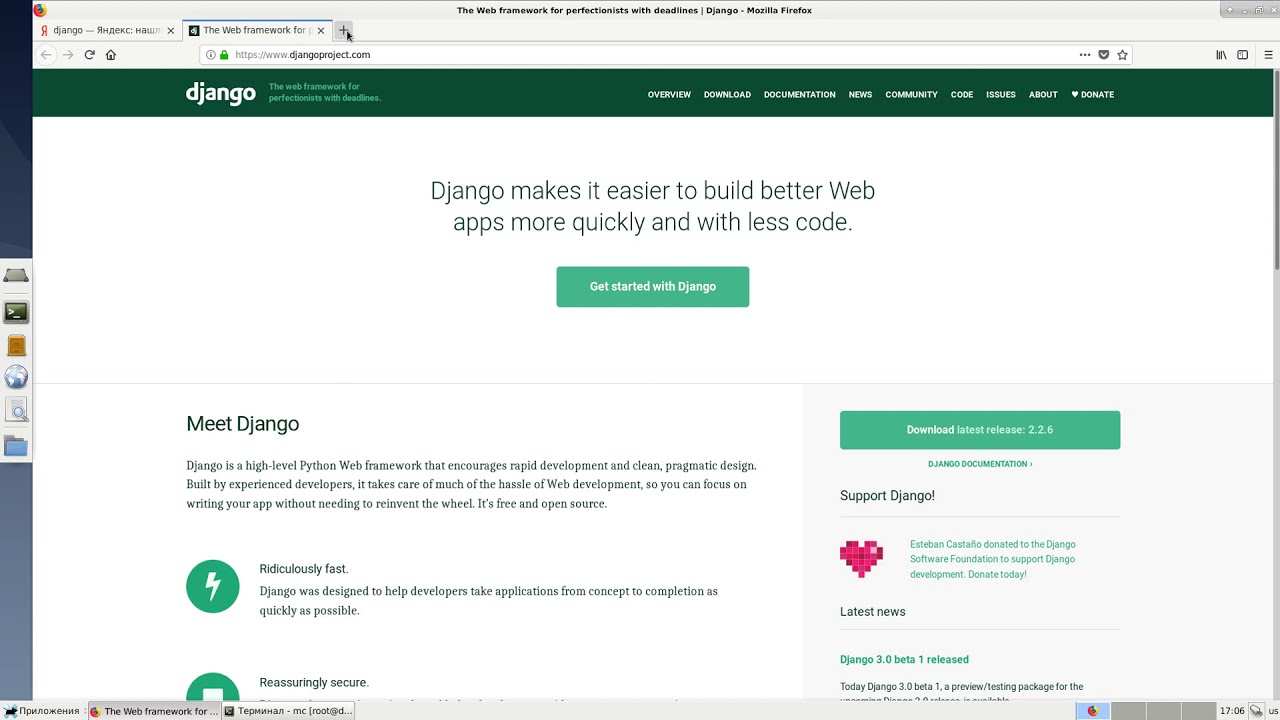**Caption:**

The screen displays a webpage dedicated to Django, the web framework for perfectionists with deadlines, accessible via DjangoProject.com. The browser is open with two tabs, one displaying "Django" alongside some text in what appears to be Russian, and the other tab showcasing the Django website.

At the top of the webpage, a green navigation bar features various sections: Overview, Download, Documentation, News, Community, Code, Issues, About, and a heart icon with a Donate link. Below this green strip, the page has a white background with green text stating, "Django makes it easier to build web apps more quickly and with less code." This message prominently emphasizes the benefits of using Django, with "Web" capitalized for emphasis.

A green button with white text inviting users to "Get Started with Django" is clearly visible. Below this is an introductory section titled "Meet Django," explaining that Django is a high-level Python web framework designed for rapid development and clean, pragmatic design. The description highlights that Django, developed by experienced developers, aims to simplify web development, allowing developers to focus on their applications without needing to reinvent the wheel. It also emphasizes that Django is free, open-source, and designed to help developers build applications quickly and efficiently.